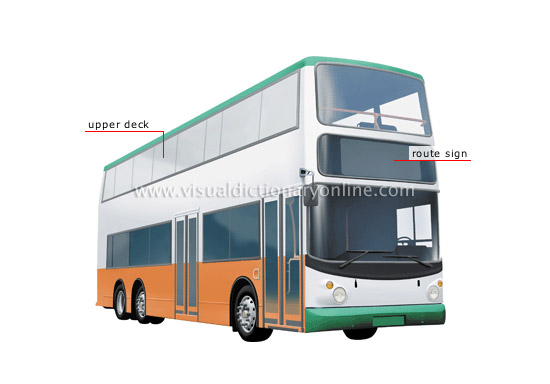The image shows a detailed, three-quarters view of a double-decker bus angled toward the right side. Most of the bus is painted white, with distinctive orange and green accents. The bottom quarter of the bus features an orange streak, while the front bumper and the roof are highlighted in light green. The bus is equipped with large, dark windows on the lower deck, and the upper deck is primarily composed of lighter, panoramic windows. Additional details include black tires, a total of three axles, and round headlights at the front. The front windshield has a route sign above it, and there's another window above the route sign for the upper deck view. A watermark reading "VisualDictionaryOnline.com" is visible, indicating the source of the image, which appears to be a computer rendering. The bus, empty of passengers, has been illustrated to provide a clear view of its design, emphasizing its spacious and modern look.